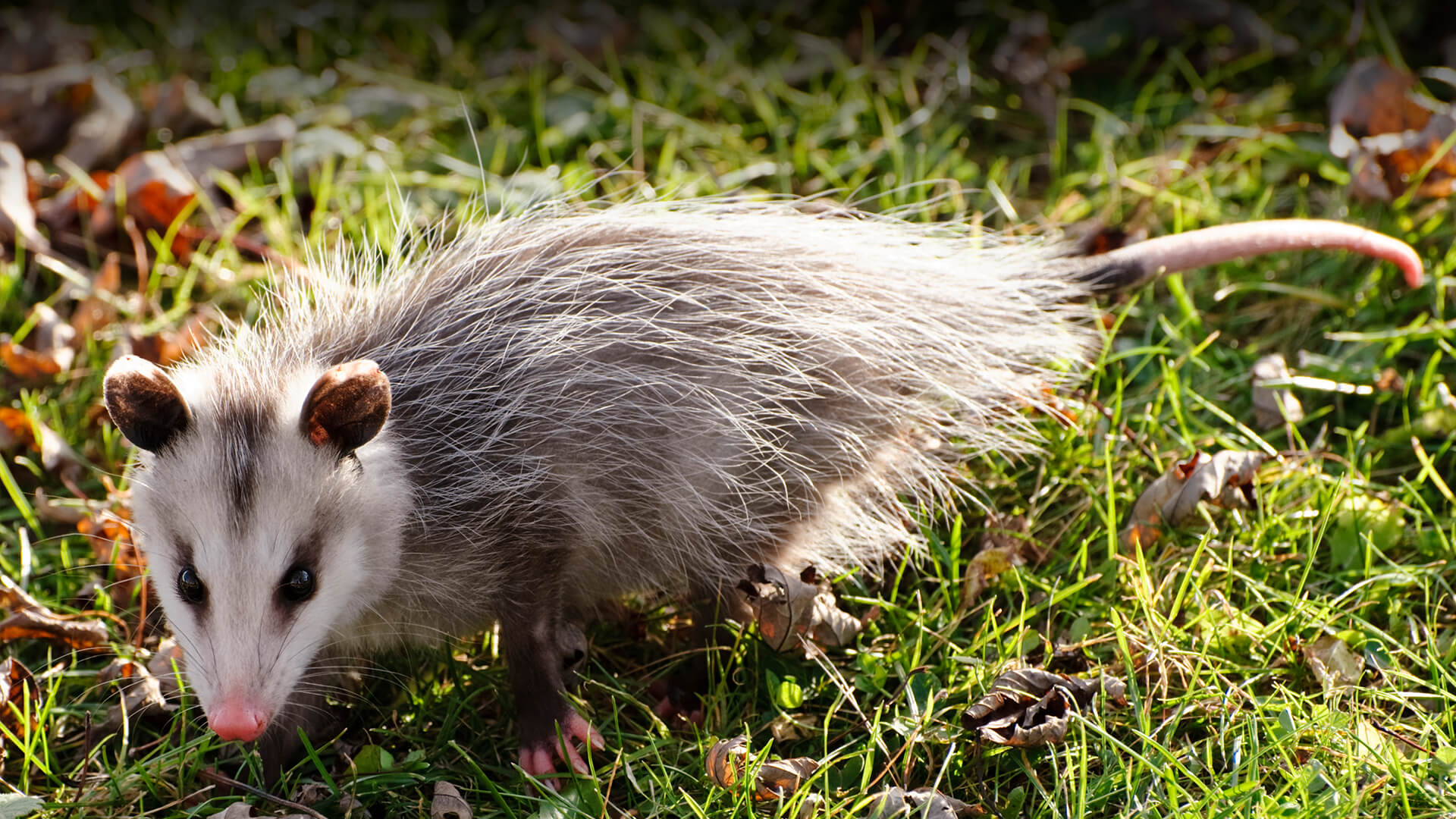In this photograph, a small opossum, likely a baby, is standing in a grassy area scattered with brown leaves, suggesting a fall setting. The green grass appears blurry in the top one-third of the image but becomes clearer towards the bottom. The opossum is positioned with its bottom to the right and its head towards the bottom left of the picture. It has a pink nose, a white face with a gray stripe down the middle, and triangular brown ears. Its large, bulging black eyes are open and seemingly looking directly at the viewer. The opossum's fur is a mix of gray and white, appearing straggly and coarse, particularly with a dark gray triangular patch on its forehead. Its delicate pink fingers and claws are visible on its dark brown paws, with at least one foot discernible. The long, skinny pink tail extends from its bottom towards the upper right side of the picture, with a slight bend at the tip. The overall composition emphasizes the opossum's detailed features and the textured, autumnal environment it inhabits.